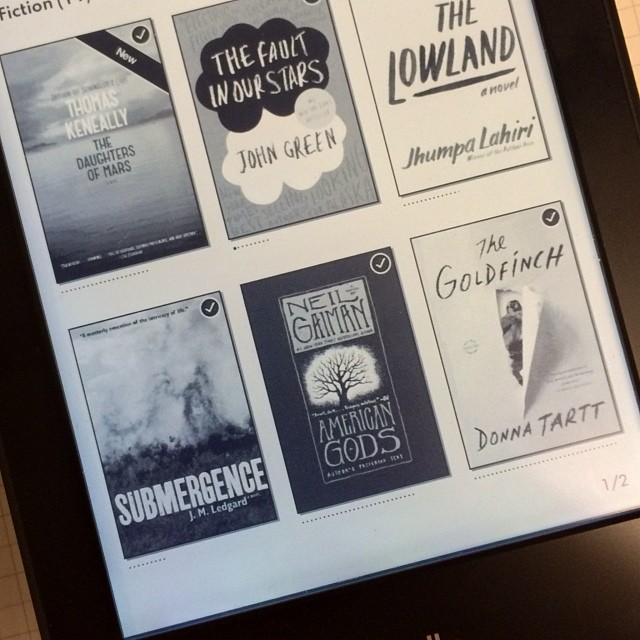This photo depicts a Kindle Paperwhite tablet displaying a library view of downloaded books. The e-reader's black bezel frames a screen that mimics printed paper, presenting black and white book covers in two rows. The first row features: "The Daughters of Mars" by Thomas Keneally, "The Fault in Our Stars" by John Green, and "The Lowland" by Jhumpa Lahiri. The second row includes: "Submergence" by J.M. Ledgard, "American Gods" by Neil Gaiman, and "The Goldfinch" by Donna Tartt. The page indicator in the bottom right corner reads "One of Two," suggesting there are more titles available. The top left corner of the screen displays the category "Fiction." The e-reader rests on a beige surface.